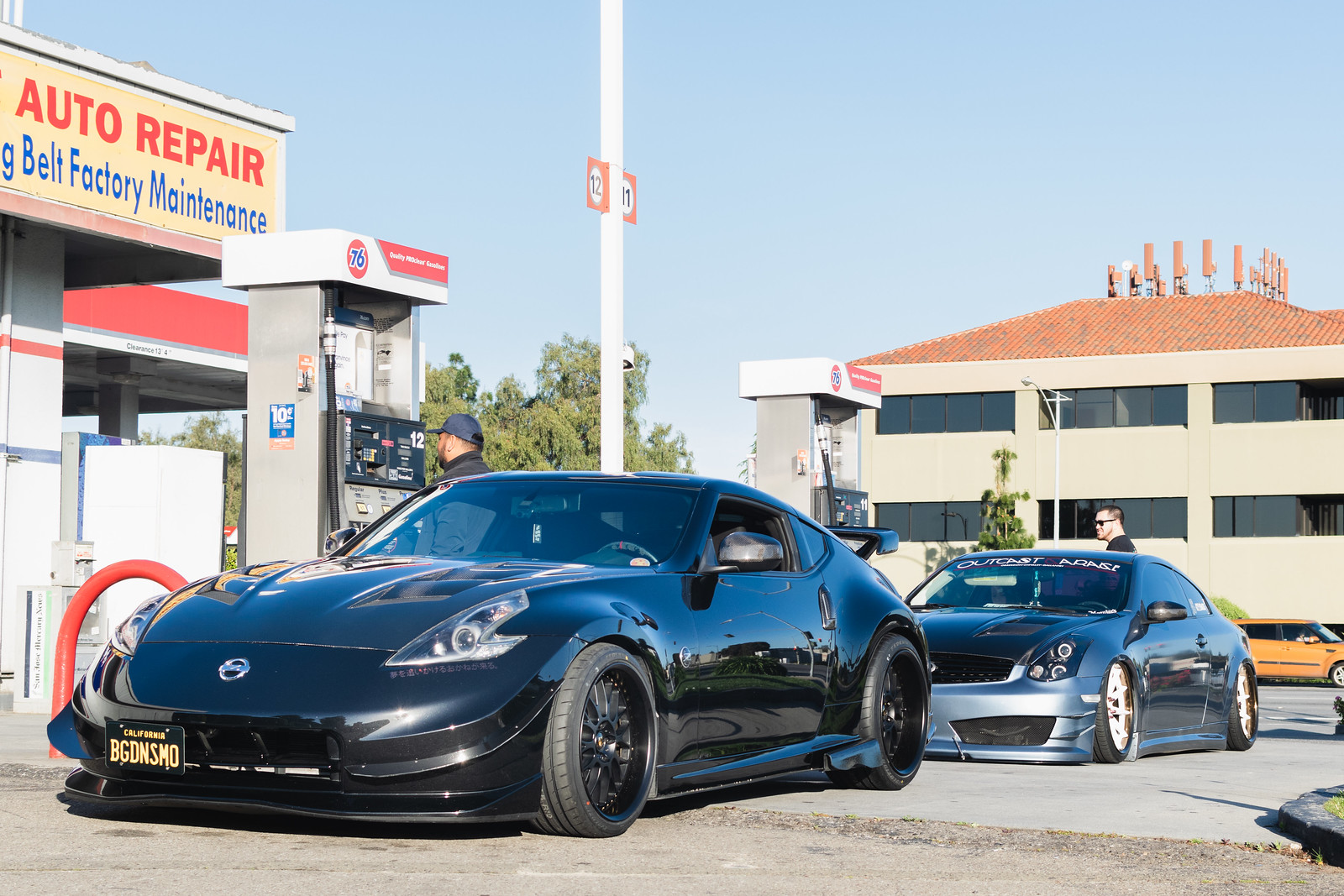The photograph, taken outdoors during the daytime, depicts a scene at a gas station, with a bright blue sky overhead. This horizontal rectangular image centers on two cars parked at gas pumps. The first car, closest to the viewer, is a black two-door vehicle equipped with a spoiler. The second car, a light gray two-door, is parked slightly behind the first. Both vehicles appear to be lowered to the ground. A gas pump stands beside each car, gray in color, and a man is visible between the pump and the black car, with only the top of his head and shoulders showing. Another man is seen standing closer to the back of the light gray vehicle.

A white pole with red squares marks the space between the two gas pumps, featuring white circles with the numbers 12 and 11 on the respective squares. On the upper left side of the image, a sign on a building reads "auto repair" in red, with "Best Factory Maintenance" in blue letters below it. In the mid-center of the image to the right, there's a beige-colored two-story building with long windows and a red-tiled roof. The cohesive elements of the scene clearly establish it as a detailed snapshot of a gas station adjacent to an auto repair shop.